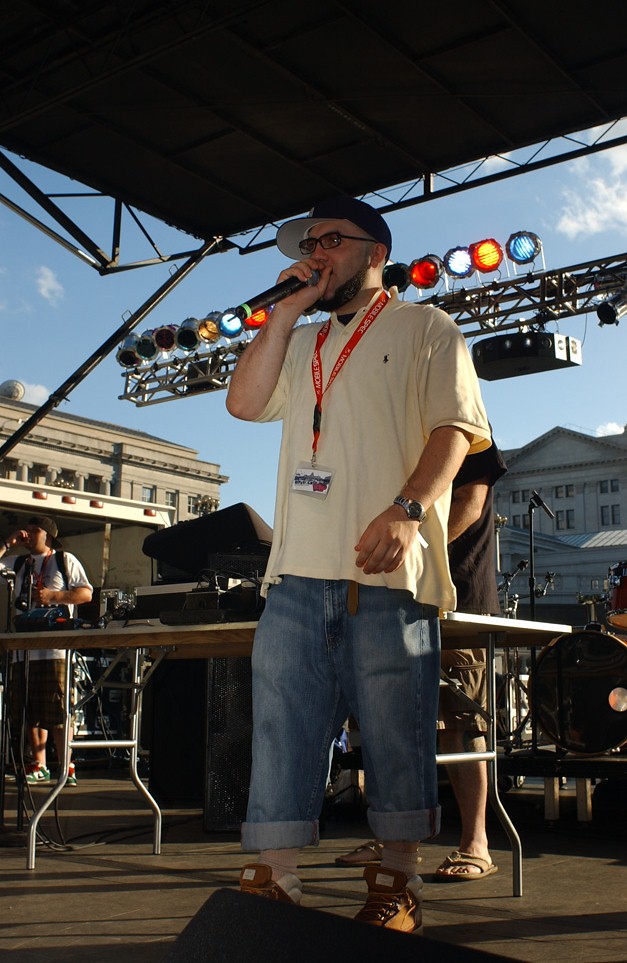The image depicts a vibrant outdoor festival or concert taking place on a bright, sunny day in a downtown area, evident from the surrounding buildings. The focal point is a bearded young man, who is possibly performing hip-hop or rap. He is standing on a makeshift stage covered by a temporary black screen tarp, which is equipped with an array of spotlights hanging from it. The performer is wearing rolled-up blue jeans, brown shoes, and an off-white or cream-colored polo shirt. He also has a red lanyard around his neck, possibly holding some credentials, and he's equipped with a microphone that is partially crammed into his mouth. His appearance is completed with a black baseball cap, plastic frame glasses, and a beard without a mustache. Behind him, there is a man, possibly a DJ, stationed at a large table with what appears to be a mixing board or turntable. The DJ is dressed in khaki shorts, a black t-shirt, and flip-flops. Additional figures are visible in the background, including some children and possible band members, although specific details about their activities or instruments are not clear. The overall scene suggests a casual, community-oriented music event with various elements contributing to a lively atmosphere.